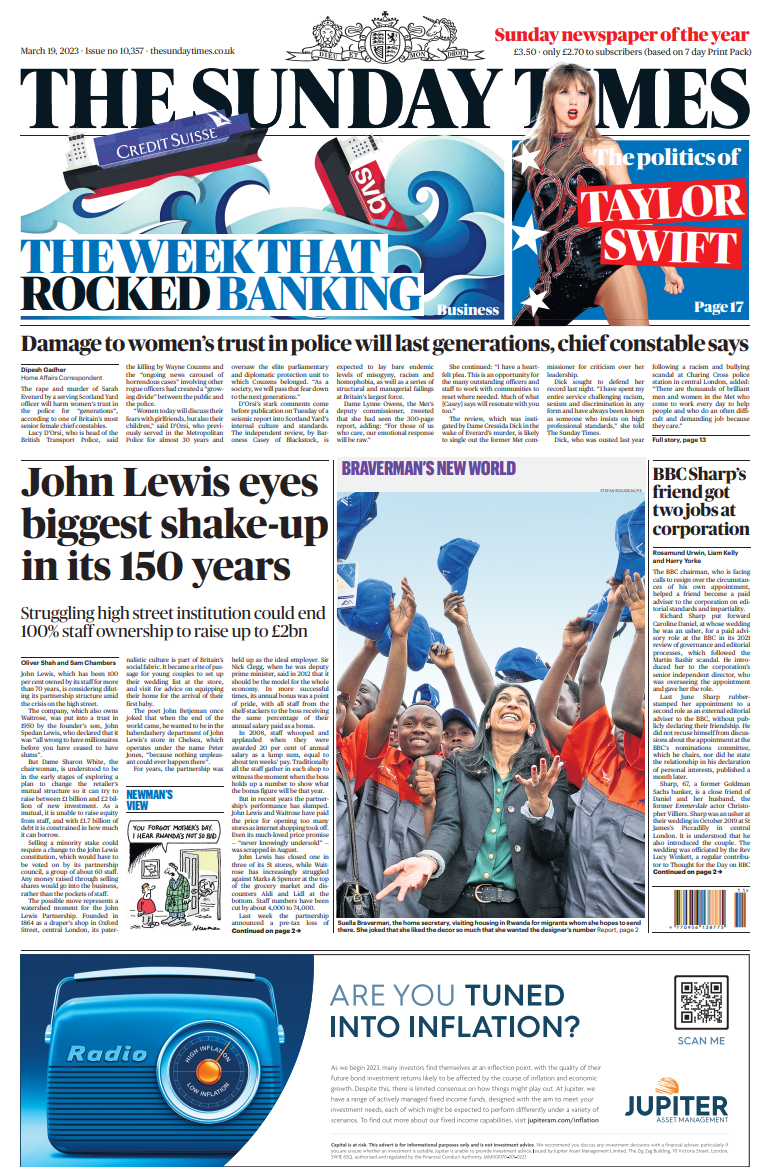This is a detailed caption for an image of the front page of The Sunday Times newspaper:

---

The front page of The Sunday Times newspaper prominently features the title "SUNDAY TIMES" in bold, black uppercase letters at the top, underlined by a regal coat of arms. The coat of arms consists of a shield flanked by a horse and a lion symbolizing strength and nobility.

On the right side of the page, there is a striking image of Taylor Swift accompanying an article titled "The Politics of Taylor Swift," exploring the pop star's influence and political views. On the left side, another prominent headline reads "The Week that Rocked Banking," illustrated with an image of tumultuous waves where cruise ships labeled "Credit Suisse" and "SVB" (Silicon Valley Bank) are depicted; SVB appears to be sinking, while Credit Suisse struggles to stay afloat.

Several other articles are featured on the front page. One headline discusses a decline in women's trust in the police, citing the perspective of a former chief constable, while another in larger text announces "John Lewis's Biggest Shake-Up in its 150 Years," signaling significant changes in the iconic retail brand. There is a photo insert showing a rally where uniformed men are celebrating by tossing their blue caps into the air, with a woman standing prominently at the forefront.

At the bottom of the newspaper, there is an advertisement from Jupiter, promoting a radio service with the tagline, "Are you tuned into inflation?"

---

This caption provides a comprehensive and detailed overview of the key elements visible on the front page of the newspaper, suitable for someone looking to understand the image without seeing it.